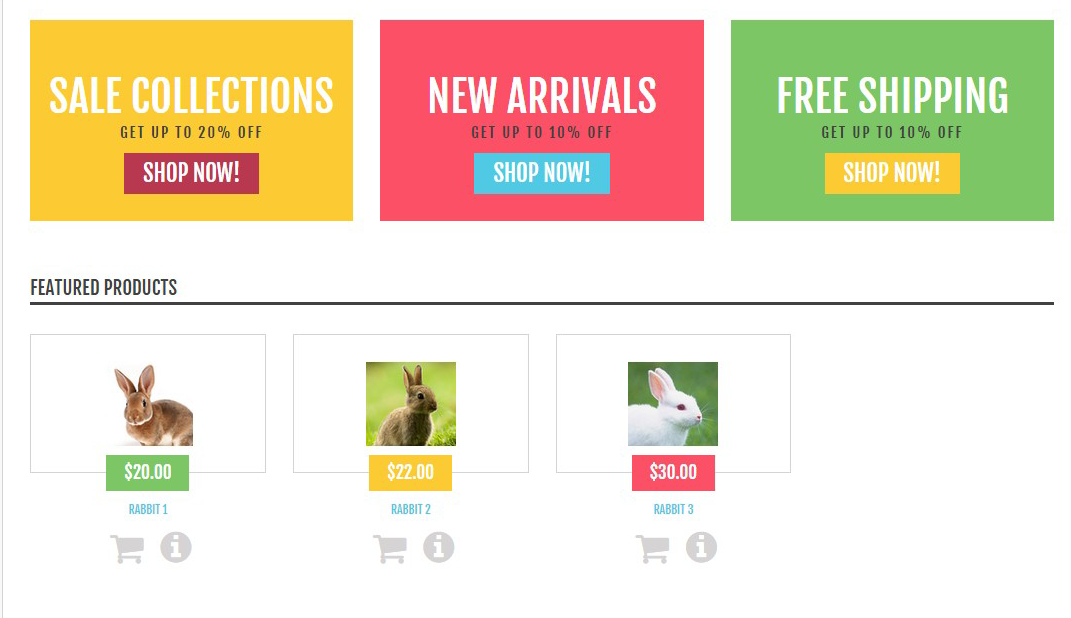**Detailed Image Caption:**
This vibrant and Easter-themed image predominantly features a white background with three prominent colored squares aligned at the top, each conveying different offers. 

- The first square, in bright yellow, announces a "Sales Collection" with a promise of "Get up to 20% off." It includes a call-to-action button that says "Shop Now!" in white text on a red background.
  
- The second square, in hot pink, promotes "New Arrivals" with a deal of "Get up to 10% off." The "Shop Now" button is styled in white text on a blue rectangular background.
  
- The third square, in bright green, highlights "Free Shipping" with a promotion of "Get up to 10% off." Again, there is a "Shop Now" button, this time in a rectangular yellow background.

Below these squares, the section labeled "Featured Products" showcases three adorable bunny toys:

- **Rabbit One:** Priced at $20, this bunny is brown with perked ears and little white paws. The "Add to Cart" icon is positioned within a small gray circle. The price is displayed in a green square.

- **Rabbit Two:** Priced at $22, this bunny is also brown, sitting upright with its ears standing straight up. It is facing sideways, presenting its big, expressive eyes. The price is displayed at the bottom in a yellow square.

- **Rabbit Three:** Priced at $30, this bunny is all white, turned sideways so only half of its body is visible. Its ears are also perked up. The price is displayed in a hot pink square.

The overall design is clean, cheerful, and visually engaging, perfect for attracting attention to the Easter-themed products and deals.